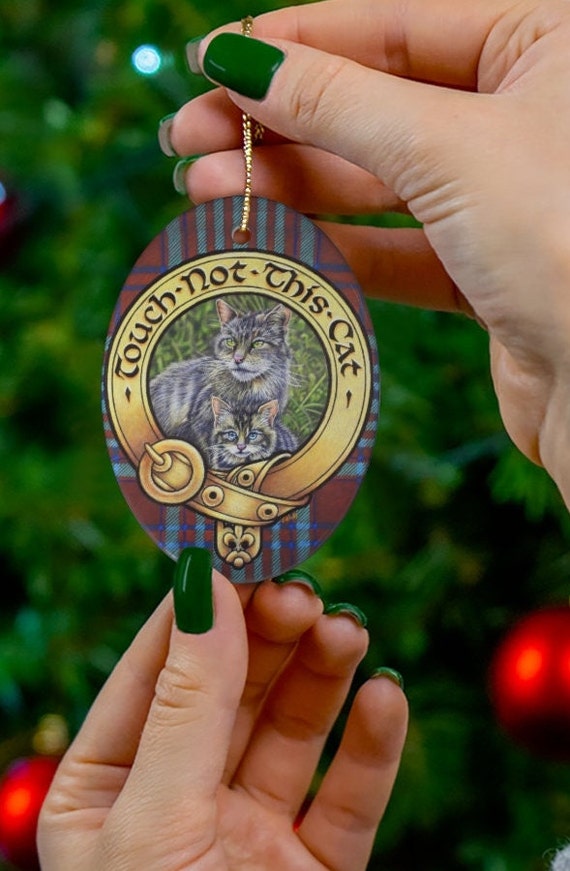In this image, a Caucasian woman's hand, adorned with green nail polish, is holding a Christmas ornament. The ornament features the text "Touch Not This Cat" and displays images of two cats on its front. There is a small hole at the top of the ornament, threaded with a string for hanging. The ornament, shaped like a belt, is decorated with a gold border. Green leaves and tree branches are visible behind the cats. In the background, a Christmas tree adorned with red ornaments is visible, indicating the ornament’s intended use as a holiday decoration.